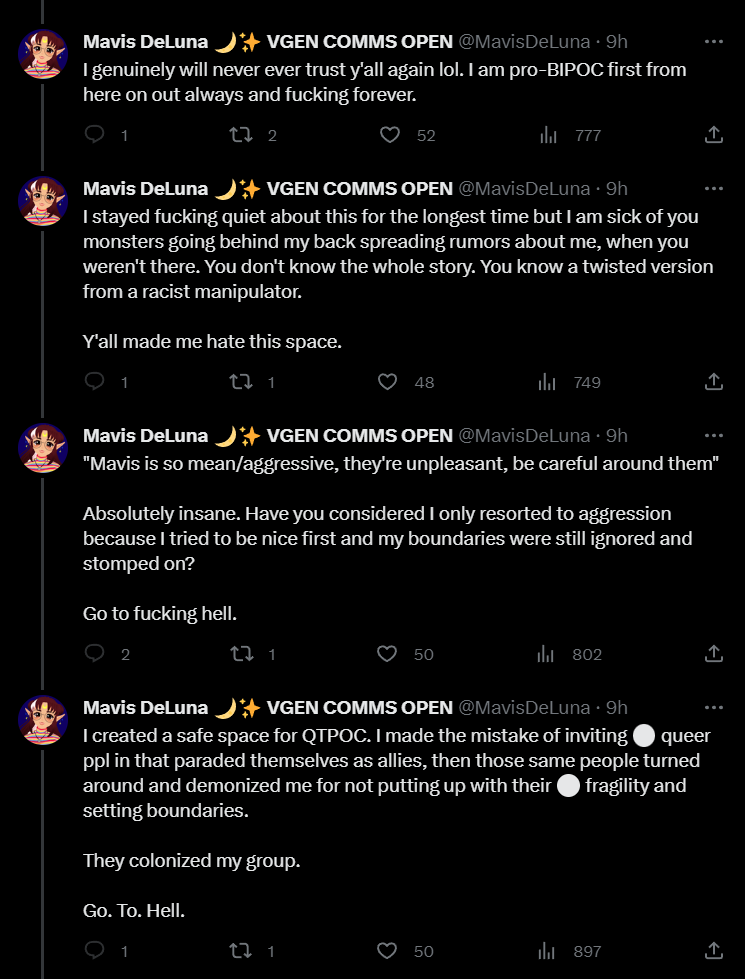This image is a cropped screenshot of a Twitter thread, likely captured on an iPad given its intermediate width—not as extensive as a desktop screenshot, but broader than a typical mobile view. The screenshot showcases a sequence of tweets and replies, all authored by the same individual. To the left of each comment, the user's profile picture is displayed, aligned vertically with a connecting line indicating the thread's flow. To the right of each profile picture is the user's name, followed by their handle in light gray text, and a timestamp showing "9 hours ago".

Each tweet in the thread appears beneath this header, with four tweets visible in total. At the bottom of each tweet, there is a series of icons: a chat bubble for comments, a retweet icon, a heart icon for likes, a bar graph icon for viewing tweet statistics, and a share icon on the far right. This layout is consistent throughout the thread. The image captures the essence of an active Twitter conversation by a single user, complete with all standard interactive elements offered by the platform.